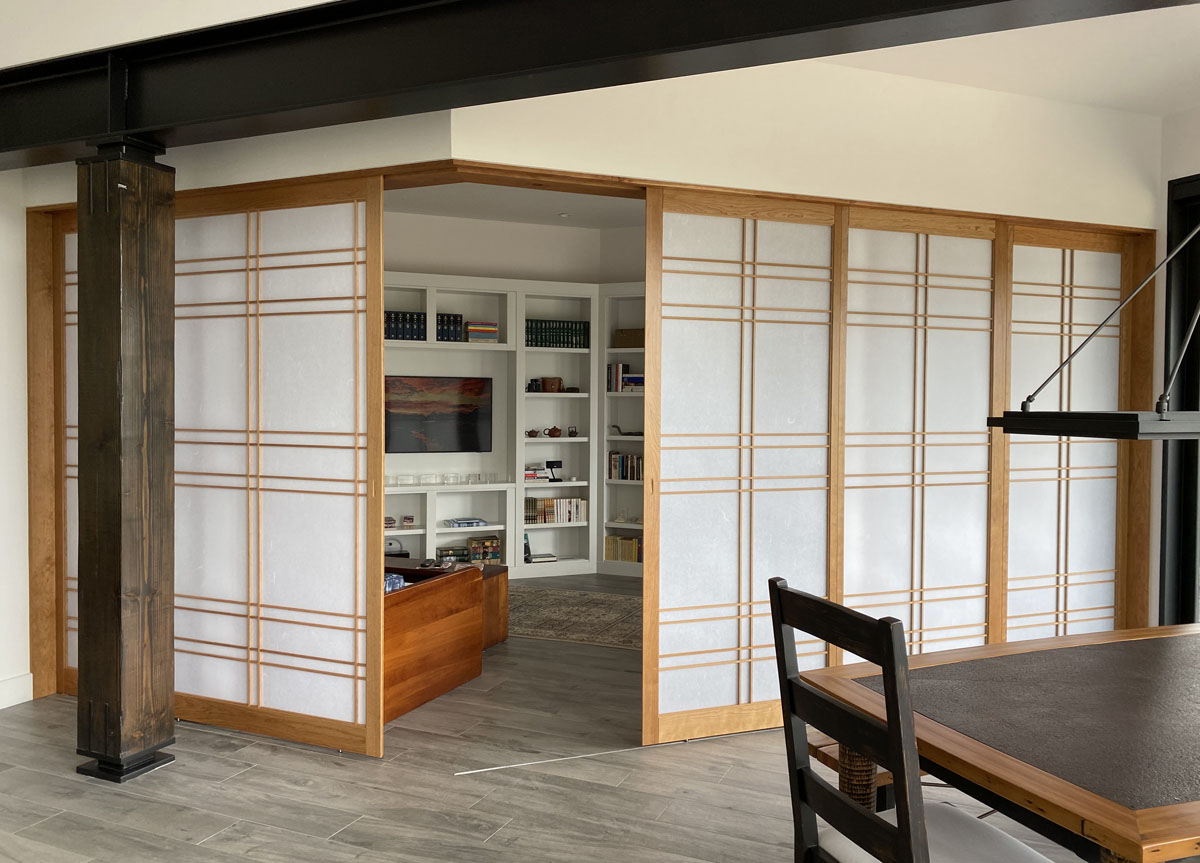The image depicts an interior space, likely inside a home, characterized by a Japanese-style design. The room features sliding wooden and paper panels, commonly seen in traditional Japanese architecture. The central focus is a living room area with dark and light shades of brown dominating the color palette, complemented by white, black, and various shades of grey. A wooden pillar supports a metal beam on the left side of the room, adding to the structural details. Shelves around a television display books, picture frames, and various decorative icons. To the right of the living room, part of a dining table and chair can be seen, extending from what appears to be the kitchen area. The walls are primarily white, but a black-framed doorway and a black pillar add contrast to the setting.